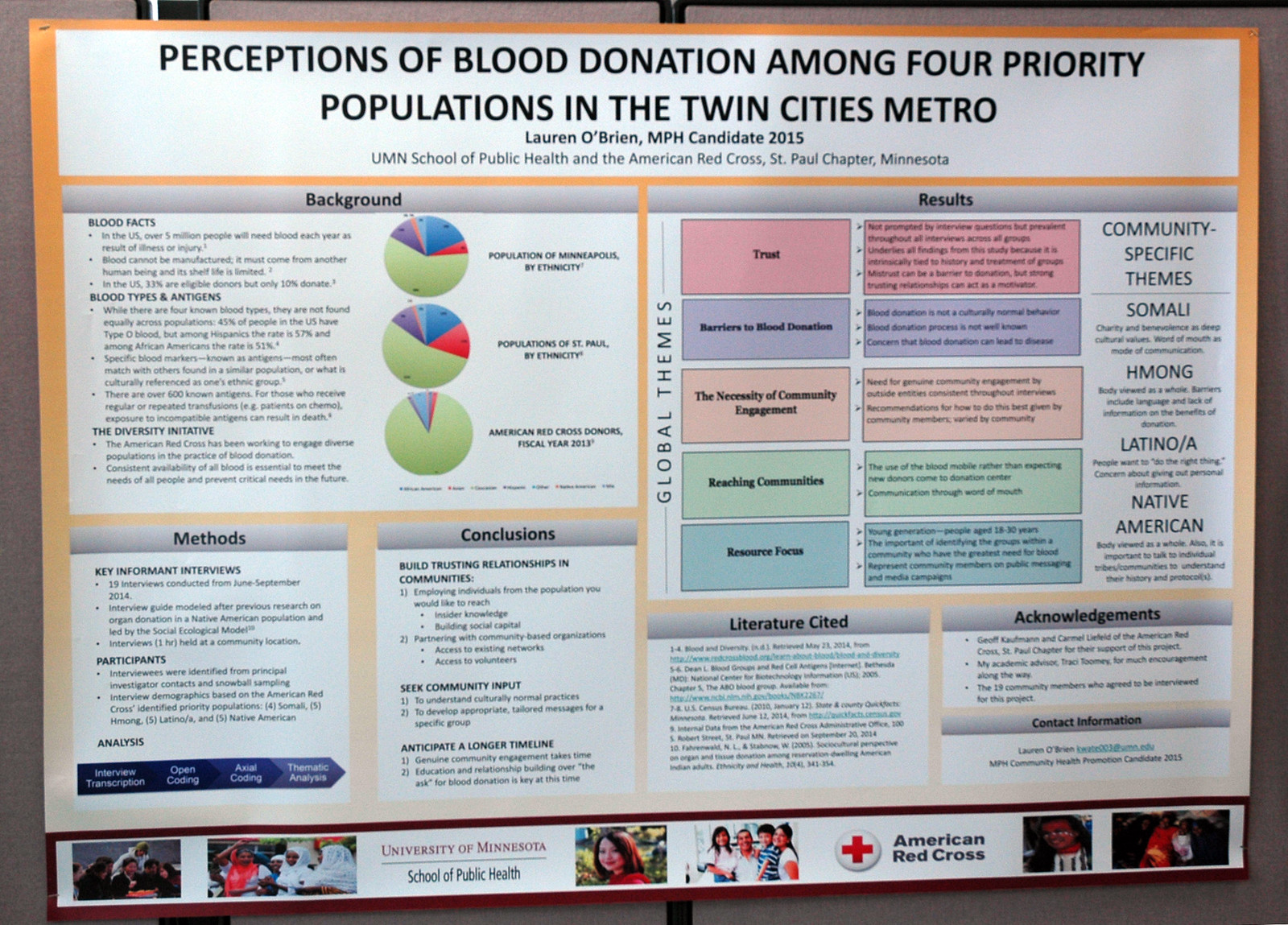The image is a color photograph of a large, landscape-oriented poster with a white background and an orange border along the top and sides. The poster features a horizontal white text box at the top with black type that reads, "Perceptions of Blood Donation Among Four Priority Populations in the Twin Cities Metro," by Lauren O'Brien, MPH candidate 2015, University of Minnesota School of Public Health and the American Red Cross St. Paul Chapter, Minnesota. The poster is divided into various sections with substantial amounts of text and data.

On the top left, there are three pie charts accompanied by text labeled "Background." The right side features columnar tables under the heading "Results," with more detailed text and colored charts depicting various testing outcomes. At the bottom left, there are two paragraphs under the subheads "Methods" and "Conclusions." The bottom right contains several paragraphs under the headings "Literature Cited," "Acknowledgments," and another heading that is illegible.

The bottom of the poster showcases the sponsors: the University of Minnesota School of Public Health on the left, along with three images of people, and the American Red Cross on the right, also accompanied by three images of people. The overall style of the poster is photographic representationalism realism.